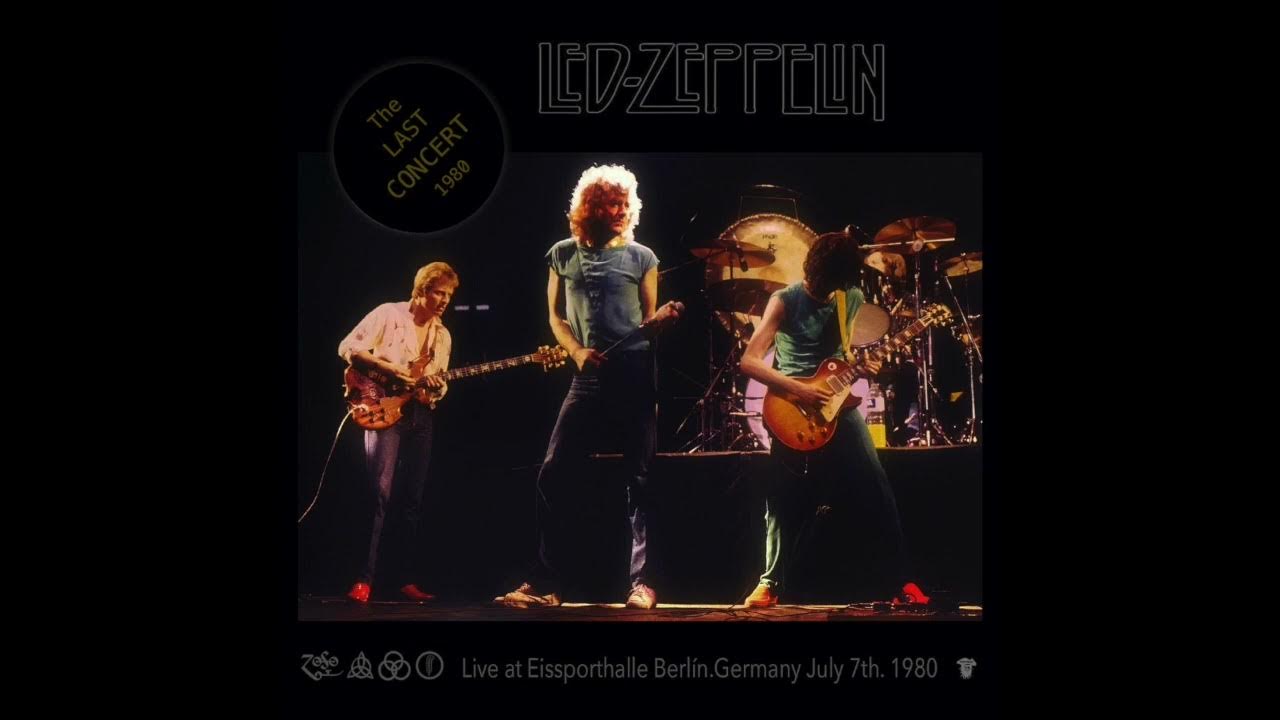The image showcases an album cover of Led Zeppelin, highlighted against a black background. At the very top, the band's name, "Led Zeppelin," is prominently displayed in white outline letters filled with black. Along the top left corner, there is a black circular emblem with a gray halo encircling it. Within this circle, the slanted yellow text reads "The Last Concert 1980," with each word on a separate line, and "Last" and "Concert" in the largest font. The centerpiece of the cover is an image of the band performing, featuring two guitarists and the lead singer at the front while the drummer is partially obscured in the back. Below this image, several white logos, including concentric circles and Venn diagram-like shapes, are visible. Beneath these logos, the accompanying text states, "Live at Eissporthalle, Berlin, Germany, July 7th, 1980." The overall palette includes varied tones—black, brown, tan, red, green, blue, gold, and gray—giving depth and vibrancy to the cover. The lead singer stands flanked by the guitarists on either side, with the drummer positioned behind the bassist, emphasizing the concert atmosphere.